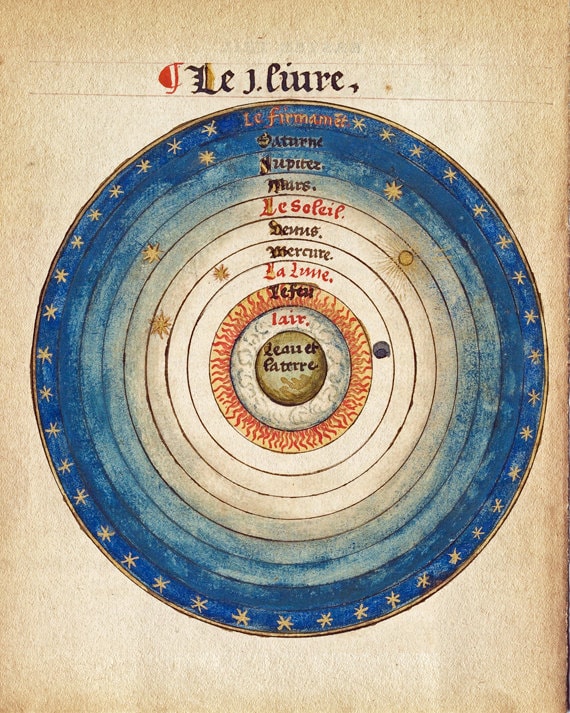This historical illustration, seemingly drawn on aged parchment, depicts an early model of the universe. At its heart, it features Earth, identified by the French label "terre," represented with a dark circular core encircled by a lighter ring possibly indicating "eau" (water). The central Earth is surrounded by concentric orbits of celestial bodies, delineated by labels in French or old Latin. Moving outward from the Earth, these orbits include the Moon, Mercury, Venus, the Sun, Mars, Jupiter, and Saturn. Beyond Saturn, the final outer circle, marked "La Fermente," signifies the realm of fixed stars at the edge of the celestial spheres. The illustration transitions from a darker blue on the periphery to gray and white toward the center, emphasizing a cosmic hierarchy. The paper, yellowed with age, features brown letters and an indecipherable title at the top. The overall circular design is enriched with layers of blue, gold, and white, encased in a thin gold border, accentuating its historical and astronomical significance.